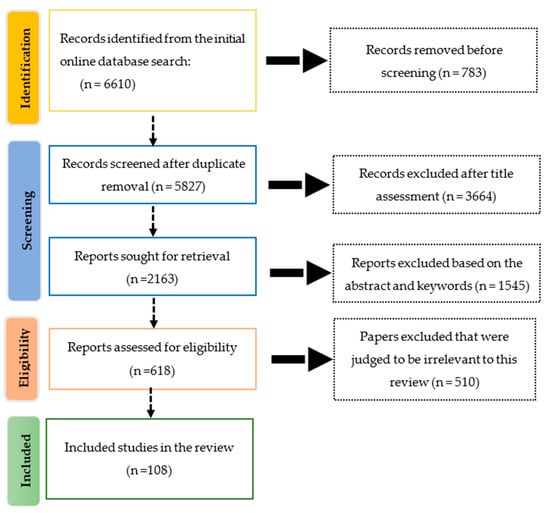This detailed infographic showcases a flowchart consisting of three columns and five main steps, visually guiding the review process of studies. On the left side, from top to bottom, five colored boxes progressively detail stages starting with a yellow box labeled "Identification" that states "Records identified from the initial online database search, N = 6,610". Below, two blue boxes are labeled "Screening". The first blue box notes "Records screened after duplicate removal, N = 5,827", followed by "Reports sought for retrieval, N = 2,163". Moving down, an orange box, marked "Eligibility", details "Reports assessed for eligibility, N = 618". Finally, the green box at the bottom labeled "Included" states "Included studies in the review, N = 108".

Arrows connect these boxes, pointing to the right where they interact with additional steps encapsulated in dotted-border boxes. These right-side stages indicate areas where records were excluded from the review process. They detail records removed before screening (N = 783), records excluded after title assessment (N = 3,664), reports excluded based on the abstract and keywords (N = 1,545), and papers excluded as irrelevant to the review (N = 510). The color-coding and organized flow of the arrows between detailed information help clarify the sequential exclusion criteria and final inclusion outcome of the review process.